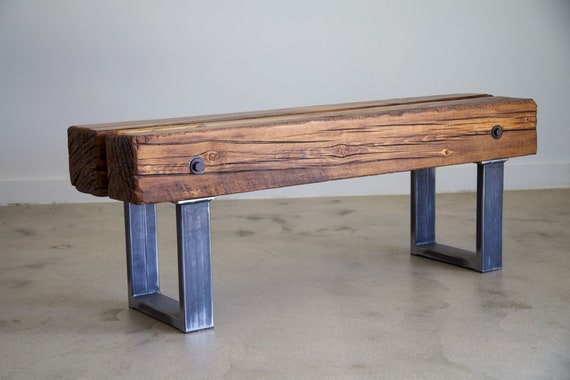The photograph showcases a small industrial-style wooden bench, possibly repurposed from rugged railroad ties. This artistic and minimalistic bench consists of two large, weathered planks of dark brown wood with visible grain lines and signs of wear and rounding. The wood pieces run horizontally, slightly angling away from the viewer from the middle left to the right of the image. The planks are securely attached by black nuts and bolts to rectangular, squared-off metal brackets or stands, which have a shiny chrome appearance. These metal brackets are bolted directly to the wood, forming a U-shaped frame that supports the bench. The setting includes a polished concrete floor with some staining, and a white wall with a white baseboard in the background. The photograph is taken at an angle, not parallel to the wall, adding to the dynamic presentation of the bench in the space.